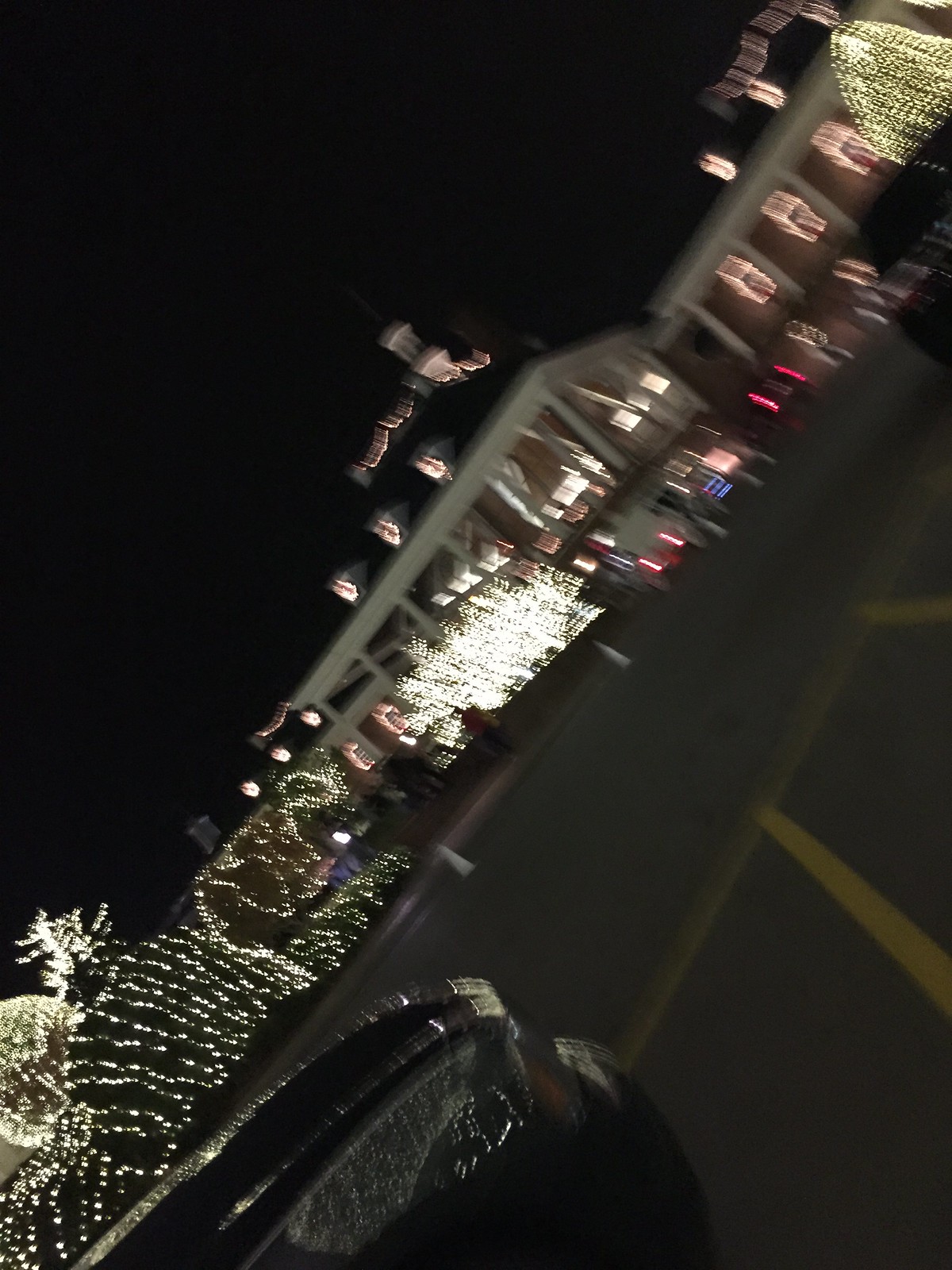Despite its blurriness, this photograph reveals a nighttime scene with several intriguing details. A black road runs through the image, bordered on the right by yellow parking lines. Part of a black car is visible, illuminated softly by Christmas lights emanating from the background. 

Dominating the scene is a large house adorned with big white pillars and an awning, adding a touch of elegance. Behind the house, a prominent tower stands tall with its windows illuminated, potentially decorated with Christmas lights. The tower's silhouette is accentuated with white Christmas lights outlining its structure.

To the front, a tree decorated with small white lights adds festive charm. Nearby, clusters of pink and blue lights could be ornamental lights on another tree or perhaps the taillights of a car, creating a colorful contrast. Another building or an extension of the same house is visible on the right, with windows aglow and a second level draped in strings of lights.

To the far left, an array of bushes and trees is adorned with vertically and horizontally strung white twinkling lights, adding to the scene’s festive ambiance. In the background, near the bottom left, a large circle of lights could be a tree densely decorated with white lights or another illuminated object. The overall blur suggests the photo might have been taken hastily, possibly from a moving vehicle.